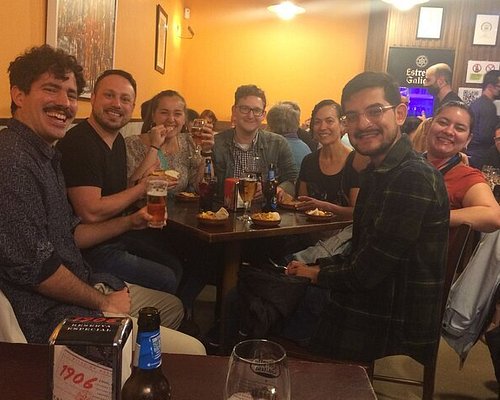The image showcases a lively atmosphere at a restaurant or bar with a group of seven friends gathered around a wooden table, all smiling at the camera. From left to right, the first person is a man with short, curly brown hair and a mustache, wearing a dark blue button-down shirt rolled up past his elbows, holding a glass of beer with his left hand. Next to him is a man in a short-sleeved black v-neck shirt. To his right, a woman in a print dress with blue, white, and brown colors is mid-bite, holding food up to her mouth with her right hand and a glass of beer in her left. Beside her, a man wearing glasses, a green sweater over a brown and white check shirt, and an undershirt underneath, is also smiling. The next person is a woman with short hair, dressed in a black top, and possibly holding a bowl on the table. To her right is a man in a green and white flannel shirt with glasses, smiling while holding what seems to be a fork or spoon in his lap. At the very edge of the table, on the far right, is a woman in a red short-sleeved t-shirt with a strap around her neck, noticeable through her short hair. The table in front of them is filled with various drinks, including bottles and glasses of beer, and a noticeable box labeled "1906" along with a bottle next to it. In the background, other patrons can be seen, adding to the bustling environment.